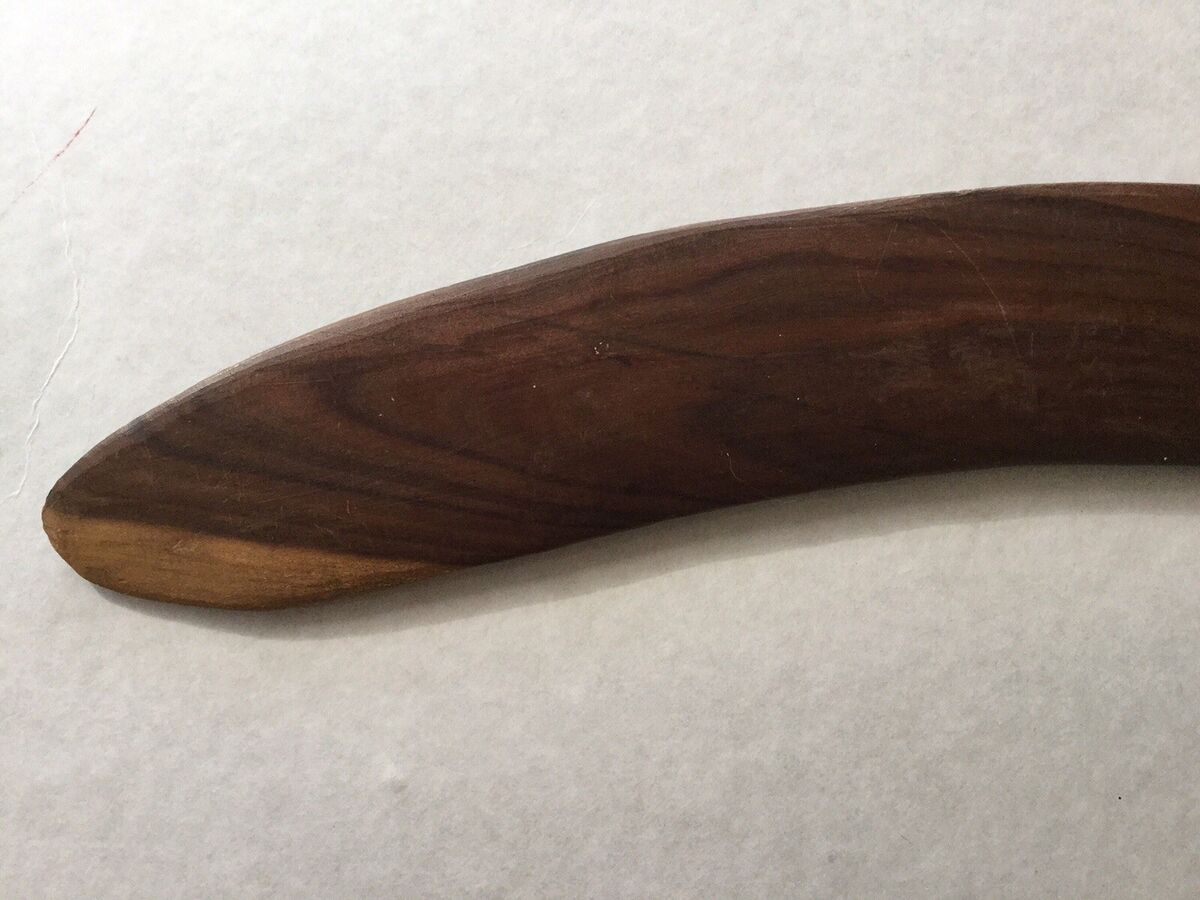The landscape-oriented color photograph features a dark brown, crescent-shaped section of wood, gracefully arcing from the top right to the left side of the image. The wood, meticulously cut, sanded, and varnished, showcases distinctive black lines and natural rings characteristic of its grain. A lighter tone adorns the rounded edge at the bottom, standing in stark contrast to the darker hues. This wooden piece rests on a white table - possibly adorned with a white and gray mottled tablecloth or rug - casting a shadow that suggests a light source is positioned above, illuminating the top left and creating a gradient effect towards the bottom right. The photograph captures the fine details of the wood and its textured background, presenting a crisp, lifelike representation of the subject.